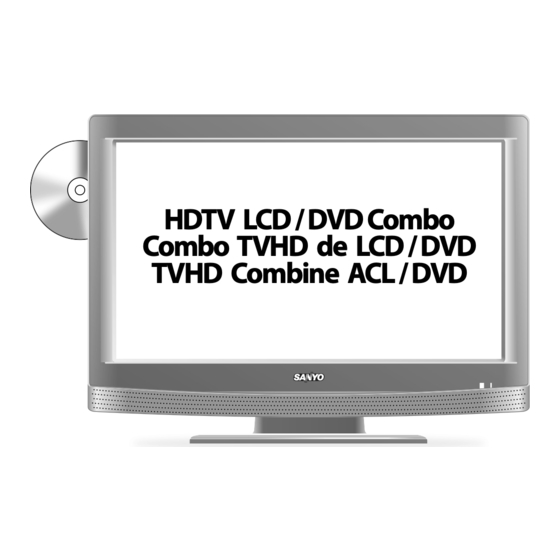The image showcases a detailed black and white drawing of a Sanyo TV, characterized by its steel gray, silvery color. The television prominently displays the brand name "Sanyo" in whitish text below the screen, accompanied by an area that appears to be a speaker grille beneath the logo. The TV is placed on a flat stand matching its color. To the top left portion of the screen, a CD/DVD is partially inserted, indicating its functionality as a combo device. The screen itself displays bold black text on a white background with three lines of information: "HDTV LCD DVD combo," "combo TV-HD DE LCD DVD," and "TV HD combined ACL DVD." Additionally, there are two light indicators on the bottom right corner of the TV.